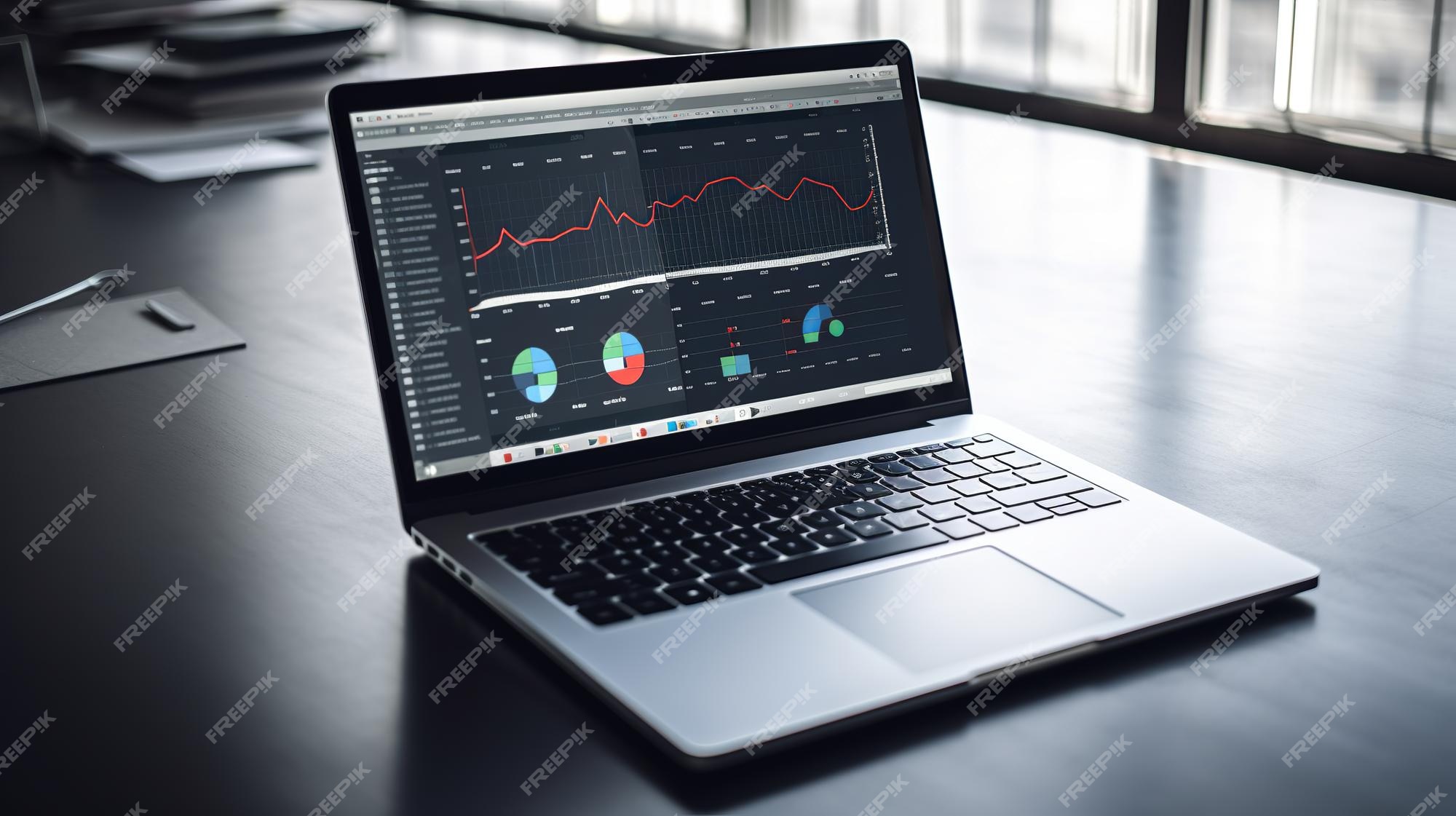The photograph captures the interior of a sunlit office or conference room dominated by a large, black table that occupies most of the image. Central to the scene is an open grey Apple laptop sitting on the table. The laptop's screen displays a dark-themed interface featuring a red line graph prominently on top, accompanied by an assortment of colorful pie charts in green, blue, and red at the bottom. The background is marked by numerous windows framed with black panes that flood the room with natural light. Additionally, clipboards can be spotted in the background. Diagonally spanning the entirety of the photograph, from left to right and top to bottom, is a conspicuous watermark that reads "FREE P!K."